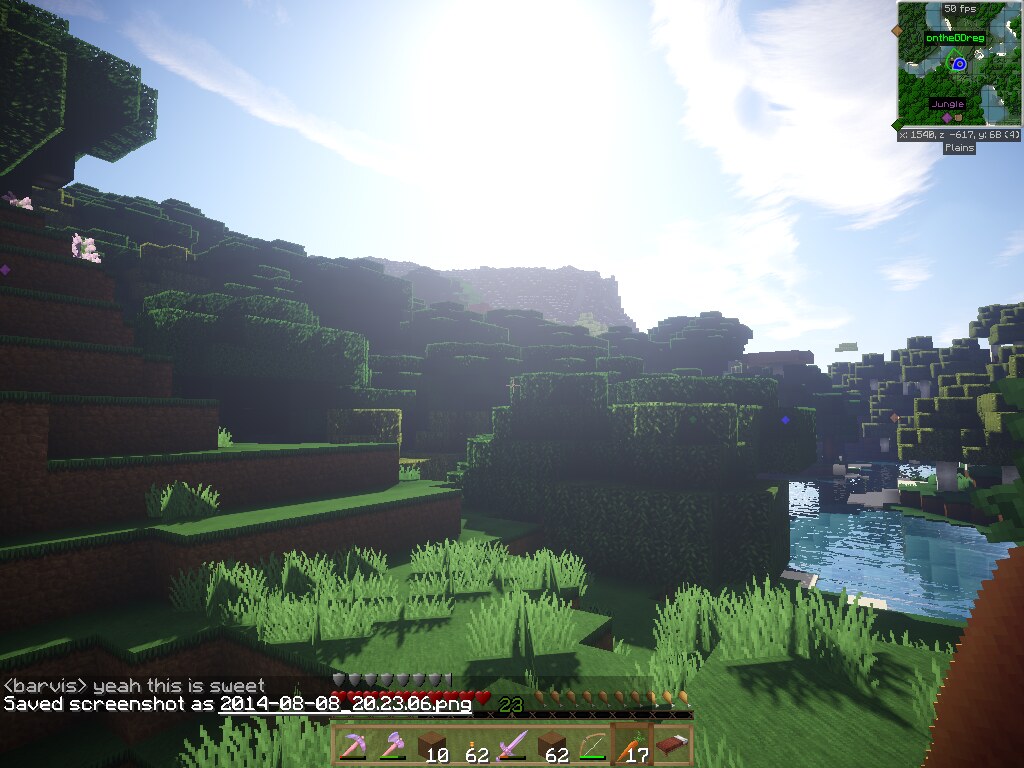This image is a screenshot from a video game, dated 2014-08-08, with the filename 2023.06.png. It prominently features a lush, green, blocky landscape with varying levels of terrain, including low-cut grass and higher tufts of grass. Block-shaped trees, or hedges, are meticulously shaped into cubes. The foreground reveals green plants, possibly rice plants, sprouting from terraced areas near a body of blue water visible on the right. The sky is blue with fluffy white clouds, having lighter, triangular streaks in the center, and you can also see the sun.

In the bottom left corner, text reads "Barvis," framed by some sort of brackets, followed by "yeah this is sweet." The image also displays elements typical of a video game interface: hearts and shields indicating health, a number 23 next to a chicken icon, and inventory slots containing items such as an axe, pickaxe, sword, and crossbow. There are additional numbers and icons, including blocks labeled 10 and 62, and 17 carats, suggesting resource counts or in-game items. The pixelated, digital aesthetic unmistakably situates this scene within a virtual game world.